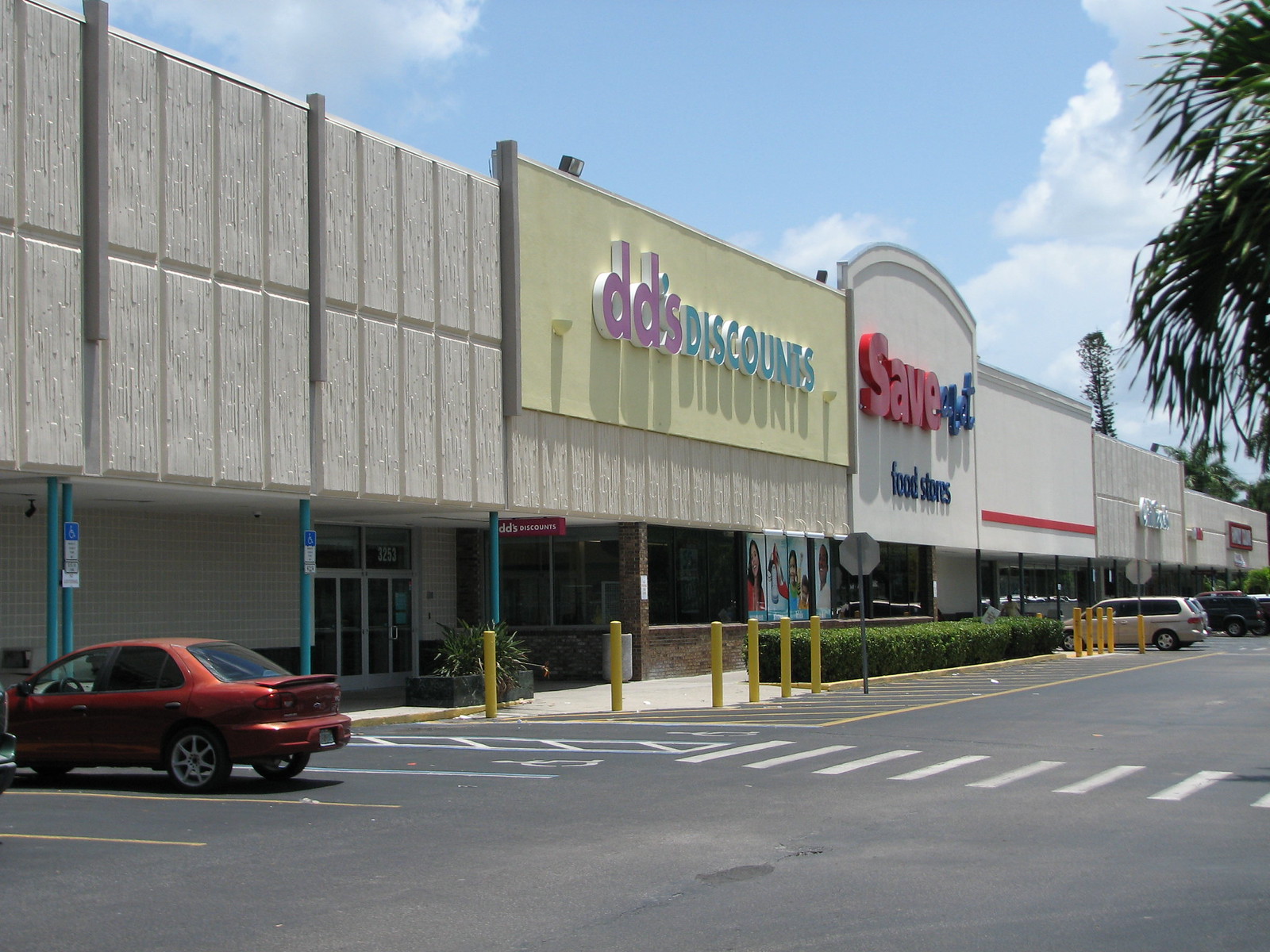The photograph captures a detailed view of an urban strip mall shopping plaza under a clear blue sky with fluffy white clouds. Dominating the scene is a prominent yellow sign for "DD's Discounts" in pink and light green lettering, central to the plaza. To the right, another large sign displays "Save-A-Lot Food Stores" in red and blue lettering. Although there are additional store signs further down the strip, they are not visible from this distance. The foreground of the image shows an asphalt parking area with clearly painted lines, including a crosswalk and two visible stop signs. Two cars, a red one to the left and a white one parked in a handicap spot to the right, are stationed in the parking lot. Along the front of the stores is a hedge and a planter box with foliage. The plaza itself features a grey upper roof and sections with a white upper roof, complemented by an overhang with supporting blue pillars, offering shelter for pedestrians. The scene is further enriched by the presence of palm tree fronds visible on the right side, and overall, the plaza exudes a typical suburban shopping environment with various amenities for shoppers.